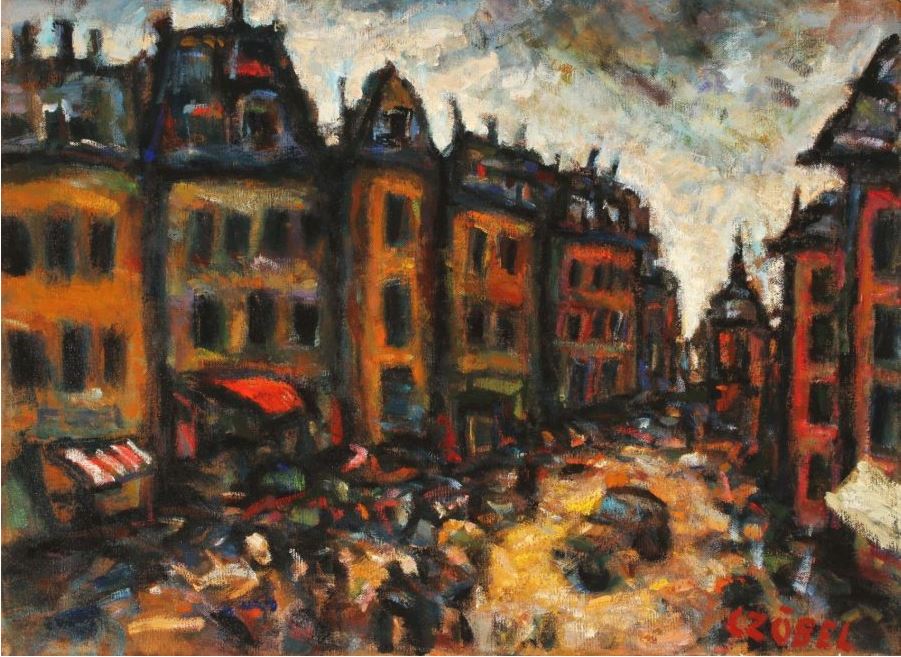This rectangular watercolor painting vividly depicts a bustling city street or public square, likely set in a European city. Dominating the left side of the painting is a row of multi-story red and orange buildings featuring tall, rectangular black windows. These structures taper inward towards the right, creating a sense of perspective. The varied rooftop designs, some triangular and others trapezoidal, all adorned with black or blue chimneys, add architectural interest.

The street, painted in a yellowish-brown hue, is lined with buildings that extend toward the right side of the image, where similar red structures are visible. The awnings on the fronts of these buildings suggest a lively street scene below, populated by abstract, colorful blobs that likely represent people. These figures, while indistinct, bring a sense of activity and movement to the composition – echoing the Impressionist style with their vibrant brush strokes.

Above, the sky features a dynamic mix of light and dark blues, accented with hints of black and other shades, suggesting day-time but perhaps with a cloudy or overcast ambience. Amid this urban tableau, the colors range from vivid reds and oranges to calming blues and greens, creating a visually striking scene.

In the bottom right hand corner, in a moderately large orange font, is the signature "Czóbel" with an accent over the 'O,' indicating the artist's name, further hinting at the painting’s European origins. The careful blend of colors and details makes this piece a fascinating representation of city life through an abstract, impressionistic lens.